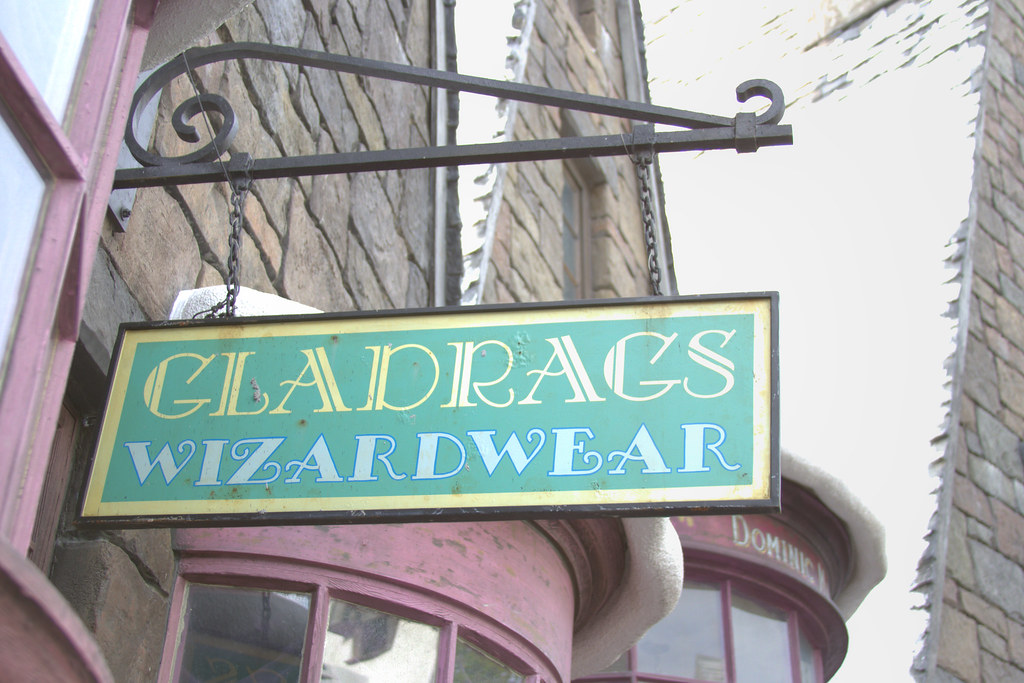The image depicts a charming shop, seemingly inspired by the Harry Potter universe, made with brown bricks and detailed with red trim. The shop features an old, elaborate sign mounted on a dark, possibly steel or black iron holder, which curls intricately at the edges. The sign, framed in a dark border, has "Glad Rags" written in yellow and "Wizardware" in white against a green background. The backdrop of the scene reveals the shop's architectural elements, including a prominent circular window with a red frame and a decorative half-oval shape, dusted with fake snow. Above the shop, the name "Dominic" is inscribed in white letters on the red portion of the building, adding to the quaint and magical atmosphere, suggesting a theme park or a whimsical setting.